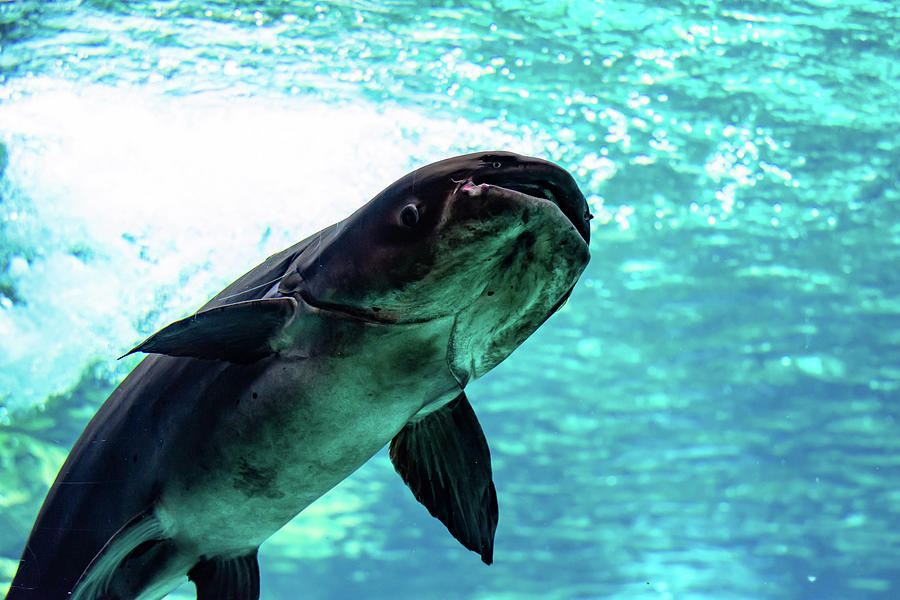This is an underwater photograph capturing a close-up of a fish, likely resembling a catfish. The fish's underside is a whitish color, contrasting its darker gray or blackish top. Both its small side fins and larger back fins are visible, though the tail is cut off by the edge of the image. The fish is oriented facing up and to the right, with prominent black eyes and what appear to be whisker-like features near its gills, which could also be interpreted as photo artifacts. The background consists of clear bluish-green water, becoming darker towards the bottom right and almost white towards the top left, suggesting sunlight filtering through the water. The image is brightly lit and very clear, emphasizing the detailed features of the fish and the serene underwater environment.